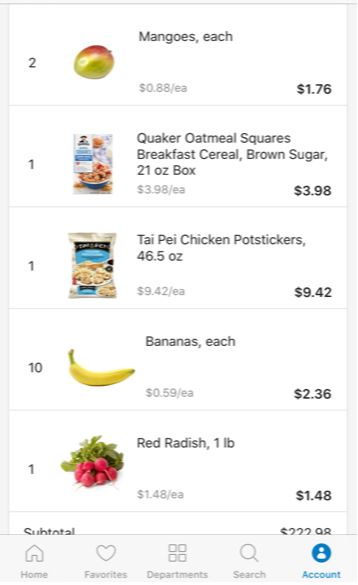This image is a screenshot captured from a smartphone displaying an e-commerce grocery website, although the specific website is not identified due to the absence of a header. The interface features a clean white background with various grocery items listed vertically. 

At the bottom of the screen, there is a navigation bar with multiple icons and labels: "Home" on the far left with a home icon, "Departments," "Favorites" marked with a heart icon, "Search," and "Account" on the far right, denoted by a blue circle with an account icon.

The grocery items in the shopping cart, listed from top to bottom, include:
1. **Mangoes:** An image of a mango is displayed, with a total price of $1.76.
2. **Quaker Oatmeal Squares Breakfast Cereal:** Accompanied by a photo of the cereal box, priced at $3.98.
3. **Taipei Chicken Pot Stickers:** A frozen meal with a blue package featuring tiny images of the pot stickers, although these details are somewhat difficult to discern.
4. **Bananas:** Represented by an image of a single banana.
5. **Red Radishes (1 pound):** Showing a photo of a fresh bunch of red radishes with leaves intact.

Each item includes an associated image and price, giving a clear and detailed overview of the user's selected groceries.